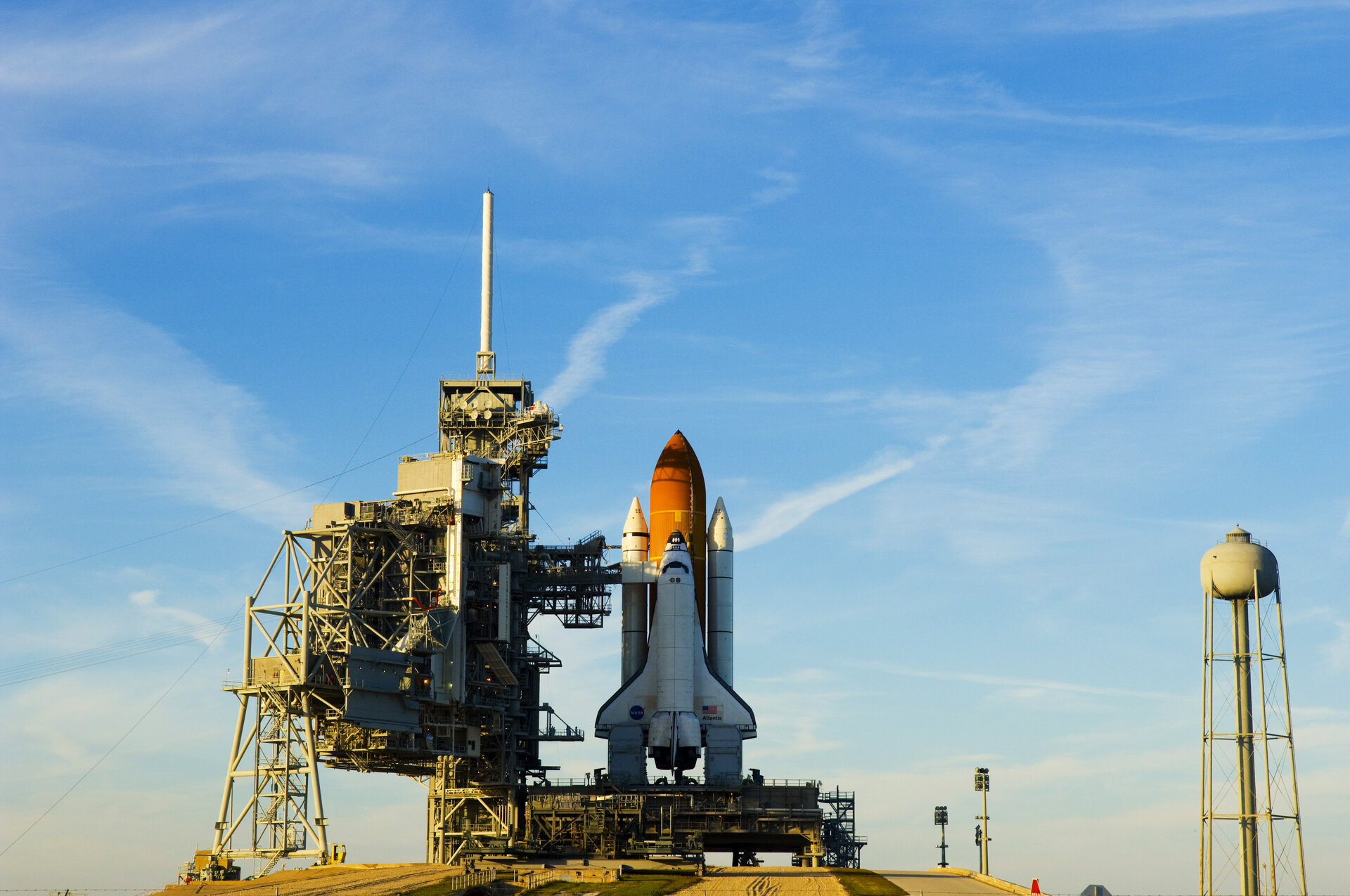This is a realistic color photograph, captured on a clear, sunny day with blue skies and scattered white clouds. The foreground prominently features a space shuttle on its launch pad, preparing for takeoff. The space shuttle, recognized by its signature white body, large red booster underneath, and two fuel tanks flanking it, is pointed upwards. It is anchored to a tall metal platform adorned with complex scaffolding and machinery, detailed in dark brown hues. A large support tower extends to the left of the shuttle, featuring connecting platforms which suggest the pathways astronauts use to board. In the background, to the right, a white water tower stands tall, adding context to the open, secluded area devoid of any people, text, animals, or vehicles. The image exudes a sense of anticipation and readiness, capturing the technical marvel of human space exploration in a serene setting.